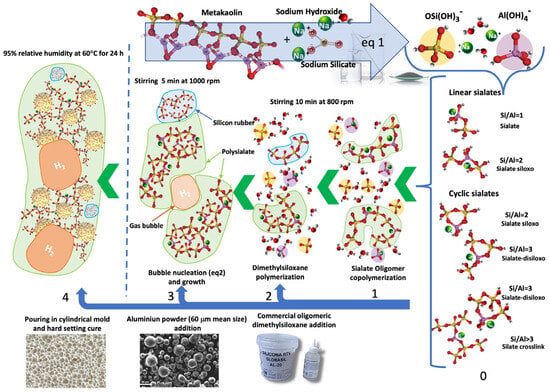This intricate horizontal image is divided into three sections, with the central portion being the most prominent. The left third features oblong shapes containing jacks-like structures and two orange blobs, numbered one through four, accompanied by four upward-pointing green arrows. Below this, there is a gray area with additional writing. The central section illustrates a series of interconnected blobs and jacks, depicting a dynamic process that resembles a cycle. This portion features several green arrows conveying movement and transformation. The image seems to illustrate a chemical or biological process involving sodium hydroxide, sodium silicate, commercial oligomeric dimethyloxane, aluminum powder, and steps like pouring into a cylindrical mold followed by hard-setting cure. The graphic includes detailed molecular structures with red, yellow, purple, and green components, demonstrating complex interactions and stages within this chemical process.